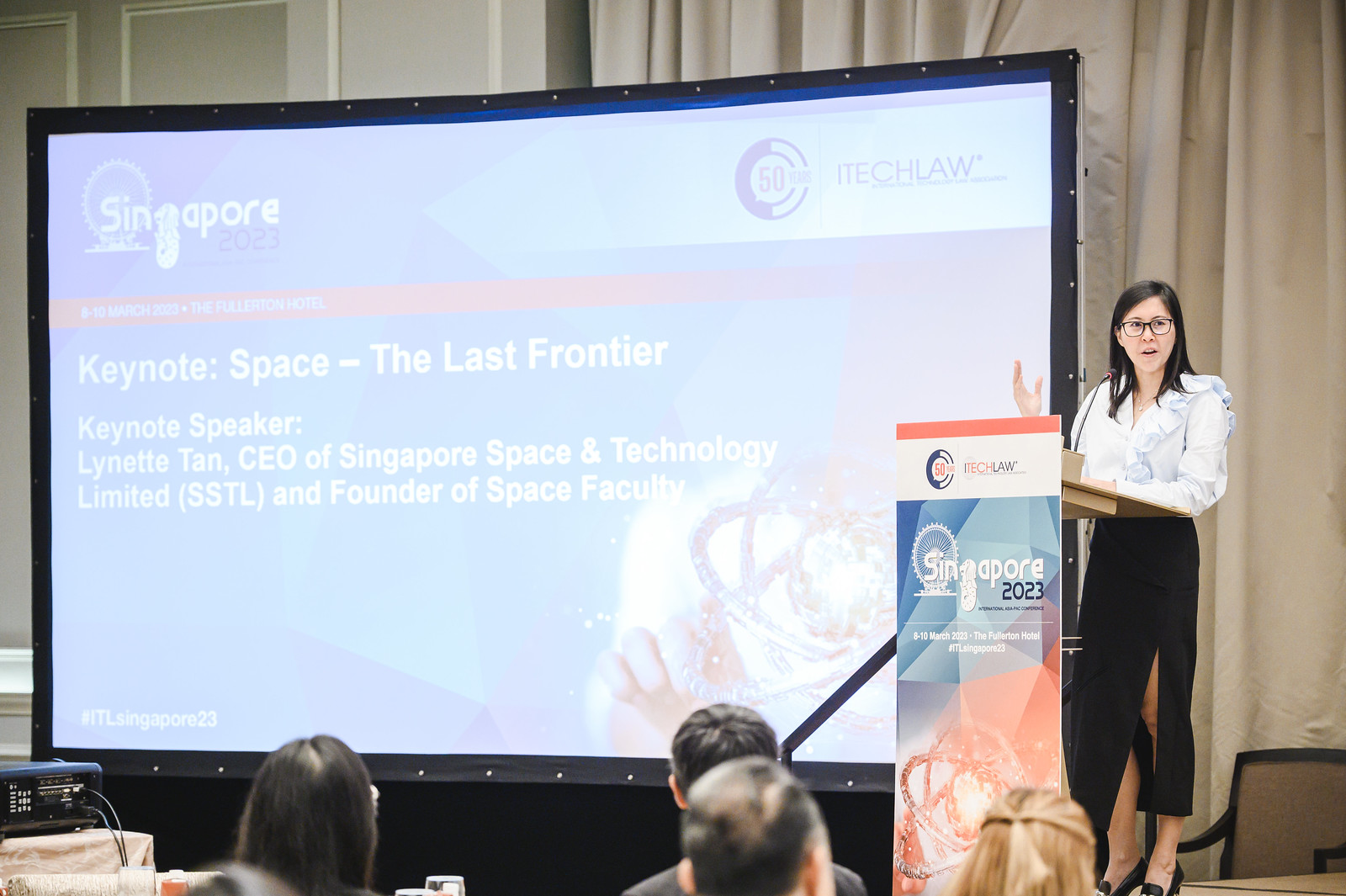In this indoor photograph of a convention or seminar, a woman, identified as Lynette Tan, CEO of Singapore Space and Technology Limited (SSTL) and founder of Space Faculty, is seen speaking at a podium. She is wearing black pants, dark shoes, a white long-sleeved blouse, and glasses. Her right hand is raised, indicating she is engaged in her speech. The podium is branded with the iTech Law logo and annotated with details such as "Singapore 2023," "8-10 March 2023," "The Fullerton Hotel," and "#ITLSingapore23." 

Behind her is a large projection screen with a geometric blue and pink background. The screen displays several texts: "Singapore 2023" on the top left, "50 years" and "iTech Law" on the top right, an orange-red band across the center with the event date, and the title of her presentation in white text, "Keynote: Space, the Last Frontier." The audience, partially visible with a few heads seen from behind, appears to be attentively watching her presentation. The setting is professional, highlighting the significance of the event and the speaker's prominent role in the space technology sector.